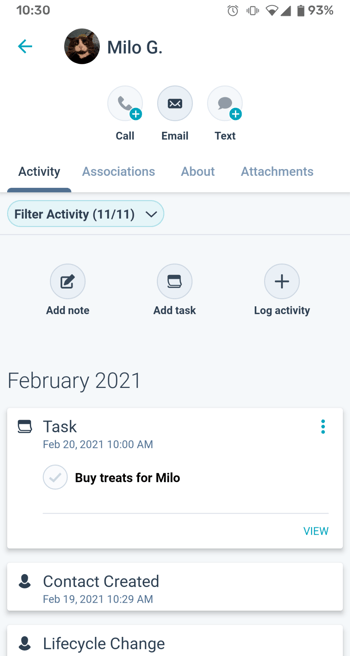A detailed image caption for a voice-generated description:

"A smartphone screen displays various notifications and task details. The time shown is 10:30 AM, with the phone set to vibrate mode and a battery level at 93%. The Wi-Fi signal is strong, showing full bars. The screen also shows several interactions related to 'Milo G,' including call, email, text, activity, associations, and attachments, all with a filter activity date of November 11. 

Additionally, the task section includes a note to 'Buy treats for Milo' scheduled for February 2021 at 10 AM, indicating a contact creation timestamp of February 19, 2021, at 10:29 AM. The screen details tasks such as adding notes and logging activities, with an overall theme of task management and contact tracking."